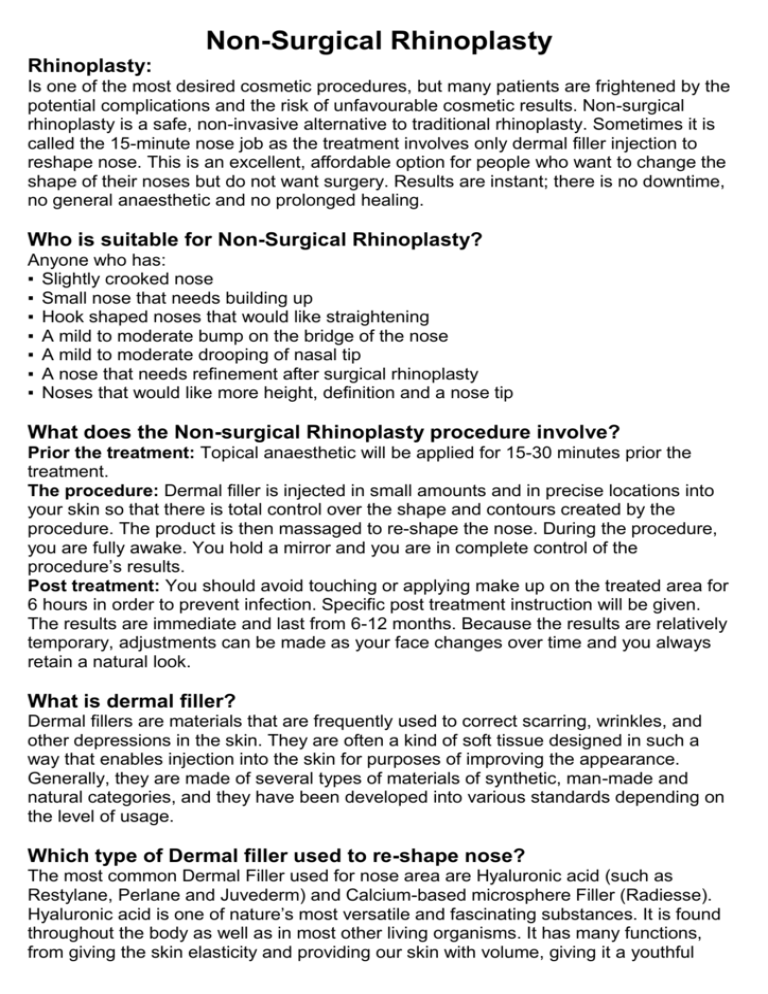**Detailed Caption:**

The image features a white page filled with black text detailing the procedure, benefits, and specifics of non-surgical rhinoplasty. The title at the top reads "Non-Surgical Rhinoplasty". The text begins by explaining that rhinoplasty is a highly sought-after cosmetic procedure, but many are deterred by the potential complications and risks associated with surgery. Non-surgical rhinoplasty, often referred to as the "15-minute nose job," presents a safe and non-invasive alternative, using dermal filler injections to reshape the nose.

The description highlights the advantages of this procedure: it is affordable, results are immediate, and there is no downtime, general anesthesia, or prolonged healing involved. Suitable candidates include individuals with slightly crooked noses, small noses requiring augmentation, hook-shaped noses desiring straightening, mild to moderate bumps on the bridge, nasal tips that droop mildly to moderately, noses that need refinement post-surgical rhinoplasty, and those seeking more height, definition, and a refined nose tip.

The procedure involves applying a topical anesthetic 15 to 30 minutes prior, followed by precise injections of dermal filler into specific locations on the nose to control its shape and contour. The filler is then massaged to achieve the desired form. Patients remain fully awake and hold a mirror to participate actively in achieving the desired outcome. Post-treatment instructions advise avoiding touching or applying makeup to the treated area for six hours to prevent infection. The results, which last from six to twelve months, allow for adjustments over time to maintain a natural look.

The text further explains dermal fillers, noting that they are commonly used to improve the appearance of scarring, wrinkles, and other skin depressions. These fillers are made from various synthetic, man-made, and natural materials, each developed to specific standards. The most commonly used dermal fillers for nasal reshaping include hyaluronic acids like Restylane, which are prized for their versatility and prevalence in the body, contributing to skin elasticity and volume. Unfortunately, the text cuts off here, leaving the final information incomplete.